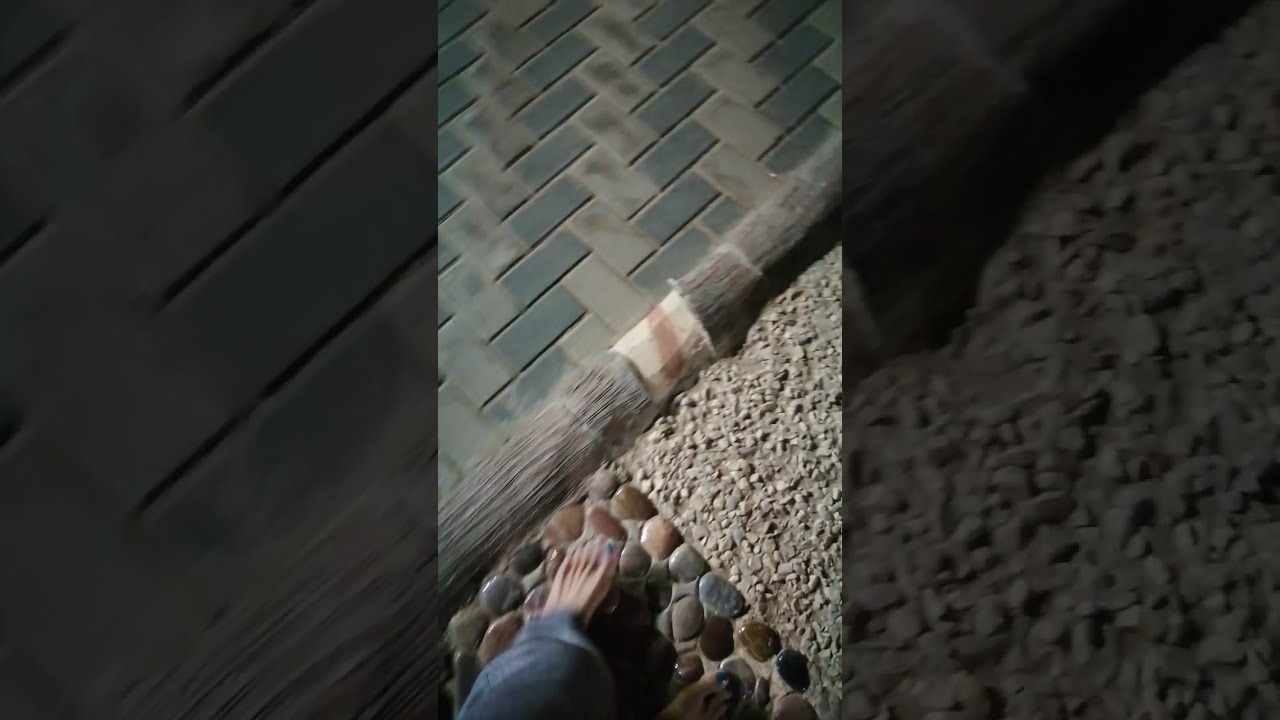The image features a downward view from just above the knee to someone's bare foot, clad in blue jeans, walking on a medium-polished stone pathway. The scene is detailed with intersecting elements: a fine gravel and pebble stone path meeting a medium- and light-gray brick path arranged in a V-pattern. There's a decorative, rounded wooden border with gray and white hues, and a brown stripe extending at a 45-degree angle, transitioning into the gravel path. The intricate flooring displays patches of tiny rocks set in concrete, forming a structured, textured surface. The main image, oriented in portrait style, appears central on the slide with two zoomed-in, blurrier close-ups on either side, set against a black opaque background, evoking a video-like format. The walking individual, possibly a woman, is captured in motion, suggesting a dynamic, real-time perspective of traversing an outdoor pathway.